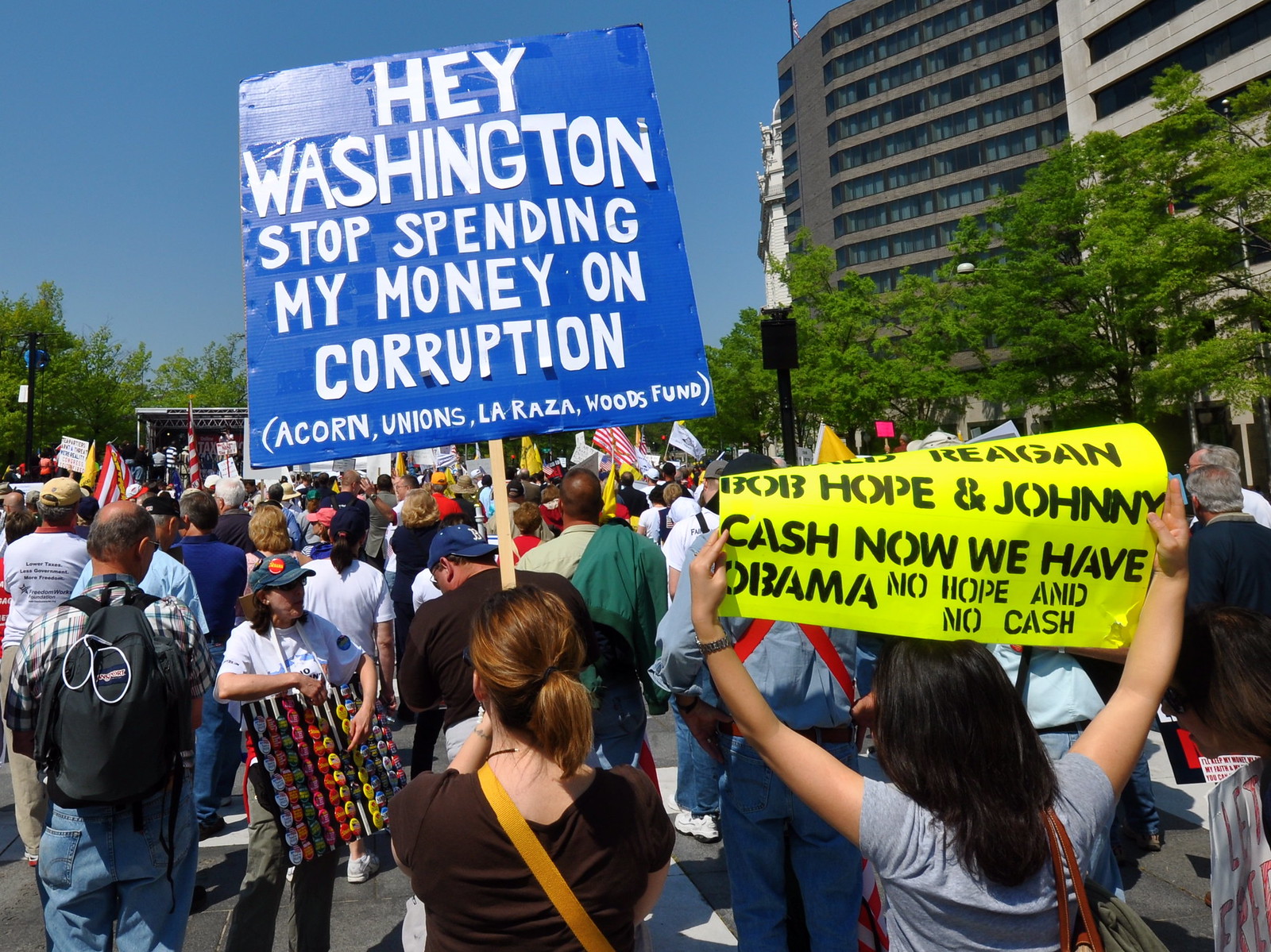In this photograph, a large crowd gathers for a protest rally in a sunny downtown park. The scene is bustling with participants, many of whom are waving American flags. Prominent among the crowd are two young women holding signs. On the lower left, a woman in a brown t-shirt with a ponytail and a yellow cross-body bag holds a blue sign that boldly reads, "Hey Washington, stop spending my money on corruption," listing "Acorn Unions, La Raza, Woods Fund." To her right, a young woman in a light gray t-shirt with a brown-strapped purse holds a neon yellow sign, slightly bent by the wind, with the message, "Reagan, Bob Hope, and Johnny Cash. Now we have Obama, No Hope and No Cash." The background features a mix of trees, big buildings with windows, and a stage set up on the left, all under a clear blue sky. The diverse crowd, mostly youthful, creates a vibrant atmosphere, indicative of collective action against government spending and corruption.